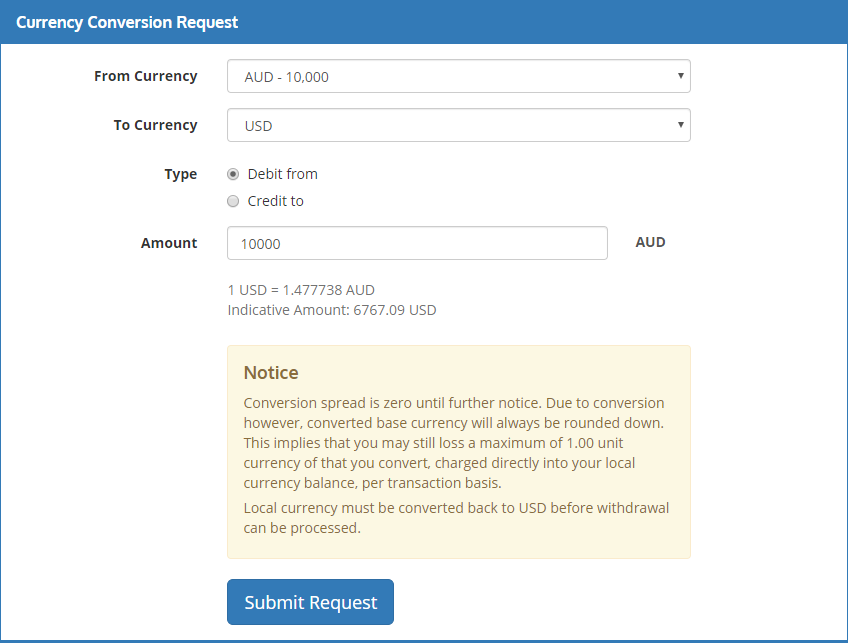The image appears to be a screenshot of a currency conversion request interface on a computer screen. The interface is framed with a blue outline and has a blue band at the top. The title "Currency Conversion Requests" is prominently displayed in white text on this blue band. 

Below the title, the interface features a white background with various text boxes and drop-down menus. The first text box is labeled "From Currency" and displays "AUD/10,000" with a drop-down arrow, indicating the user can select from other currencies or amounts. Adjacent to it, another text box labeled "To Currency" shows "USD" also accompanied by a drop-down arrow.

Further down, there is an option to select the transaction type, with two radio buttons labeled "Debit From" or "Credit To." Currently, "Debit From" is selected, specifying that 10,000 AUD will be debited. Accompanied by this, the conversion details are provided, stating that 1 USD equals 1.477738 AUD, resulting in an exchange amount of 6,767 USD for the given AUD amount.

A special notice is displayed below these details, set against a beige background with brown text, providing additional information or warnings relevant to the transaction.

At the bottom of the interface, there is a "Submit Request" button in white text on a blue background, allowing the user to proceed with the currency conversion request.